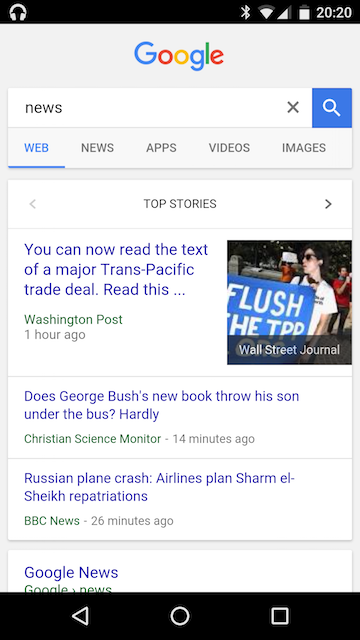The image is a cellphone screenshot displaying a Google search result page. The background of the image is predominantly light gray. At the very top, there is a thin black bar containing various icons: a headphones symbol on the left, and on the right, symbols for Bluetooth, signal strength, Wi-Fi strength, battery level, and the time, '20:20'. 

Below this bar, centered, is a Google logo illustrated in a sequence of colors (blue, red, yellow, blue, green, red). Beneath the logo, there is a white search bar with the word "news" typed in it. To the right of this search bar is a small 'X' icon for clearing the search term and a blue button with a magnifying glass icon to initiate the search.

Further down, the page has a gray background where navigation tabs for 'Web', 'News', 'Apps', 'Videos', and 'Images' are listed. The 'Web' tab is highlighted in blue, indicating that it is the active tab. Below these tabs is a small gray margin followed by a white box, labeled 'Top stories' in dark gray centered text. There are arrows on either side of the 'Top stories' heading for navigating through different stories.

The first story headline reads: "You can now read the text of a major trans-Pacific trade deal. Read this..." from The Washington Post, accompanied by a thumbnail image of a person holding a blue sign with "Flush the TPP" written in white. This is separated from the next story by a thin gray line.

The second headline reads: "Does George Bush's new book throw his son under the bus? Hardly," from The Christian Science Monitor. This is followed by another thin gray line.

The third headline reads: "Russian plane crash. Airlines plan Sharm El Sheikh repatriations" from BBC News. Another small gray gap follows before another white box that lists 'Google News' and 'Google News' in green text beneath it.

At the bottom of the image is a black banner containing navigation controls: a white triangle pointing left on the left-hand side, a white circle in the middle, and a square shape on the right-hand side.